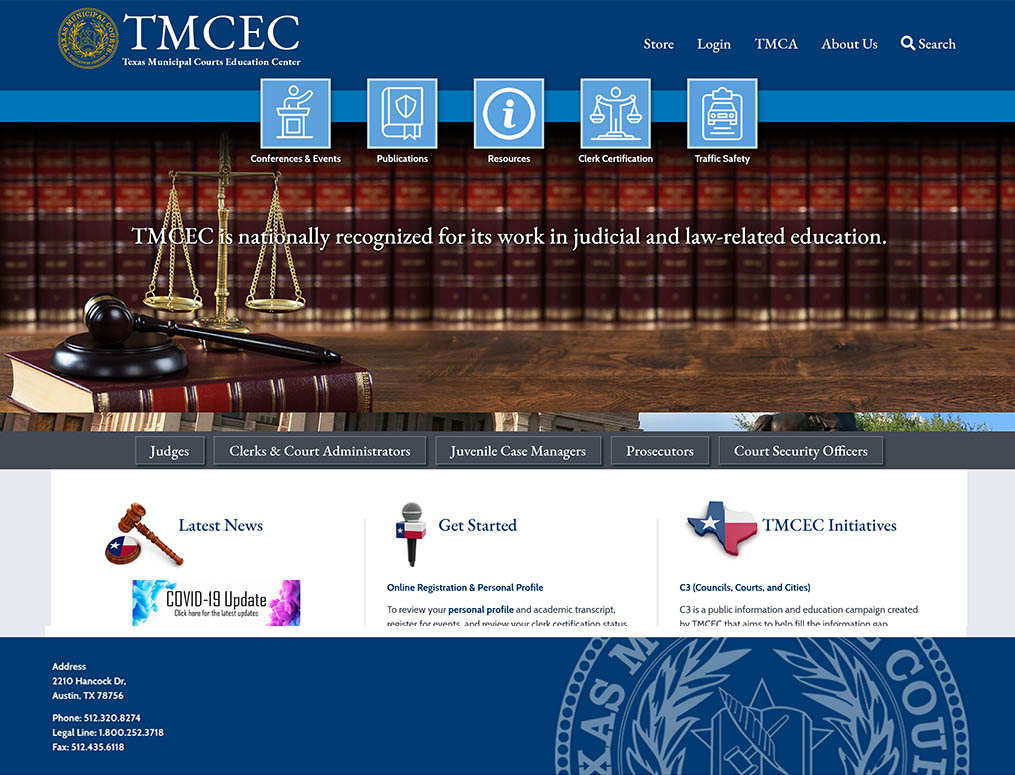This is the homepage of the Texas Municipal Courts Education Center (TMCEC) website. To the left of the TMCEC initials is the yellow official seal of the Texas Municipal Courts. At the top of the webpage, there are five navigation tabs labeled "Store," "Login," "TMCA," "About Us," and "Search." Below these tabs, five infographics highlight various functions of the website, including information about conferences and events, available publications, resources, clerk certification, and traffic safety. Dominating the webpage is a large banner featuring a photograph of a wooden gavel resting on a circular base, placed atop what appears to be a law book. In the background of the image are golden scales of justice and a row of law books, symbolizing the legal focus of the website.